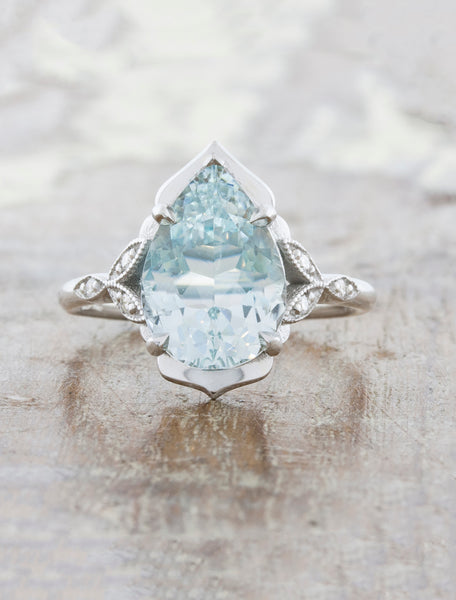A close-up photograph showcases a large, ornate ring sitting on a rough, potentially wet, grayish wooden surface. The ring is crafted from silver, white gold, or platinum, with a central light blue, clear teardrop-shaped stone commanding attention. Surrounding this prominent gemstone are intricate details: two sets of leaves encrusted with small, sparkling diamonds that flank the main stone. The lighting suggests the scene might be outdoors, enhancing the ring's reflective qualities and casting a defined shadow on the wet-looking surface. The overall effect is of a strikingly large and visually impressive piece, possibly meant as a wedding or engagement ring.